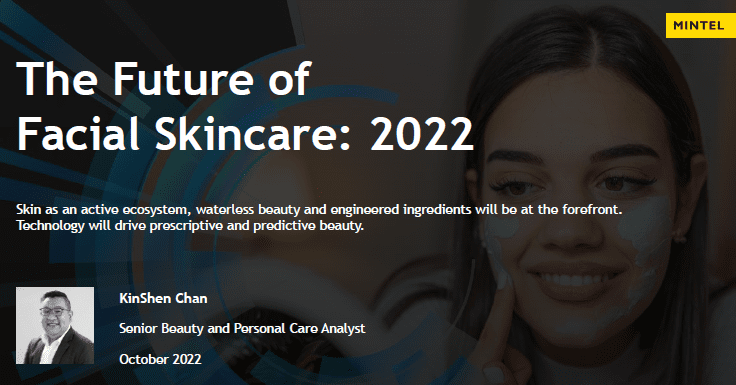In the background of the image is a woman with medium-toned skin, brown hair, and brown eyes, smiling as she applies a light blue-gray skincare product, possibly a lotion or mask, to her face. Central to the image is a promotional layout with the title "The Future of Facial Skincare 2022" in white letters. A highlighted text block details upcoming trends: "Skin as an active ecosystem, waterless beauty, and engineered ingredients will be at the forefront. Technology will drive prescriptive and predictive beauty." In the top right corner, there is a yellow box with the word "Mintel" in black letters. At the bottom left of the image, a black and white photo features Kenshin Chan, identified as the Senior Beauty and Personal Care Analyst, dated October 2022. Chan, presumably of Asian descent, is smiling and wearing glasses.